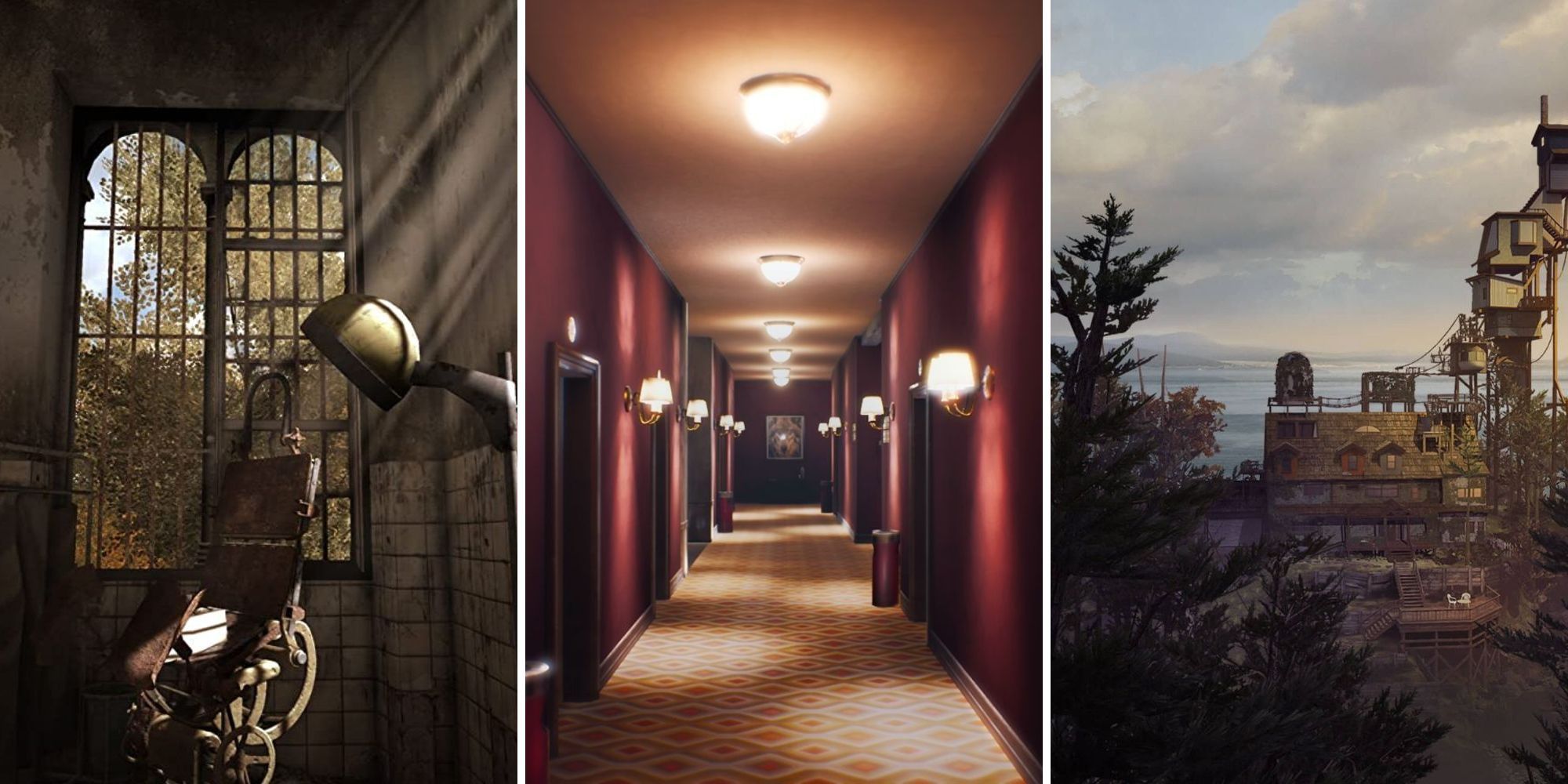This striking collage consists of three distinct photographs that showcase different environments and settings. The first image on the left captures the eerie interior of an abandoned, dingy room that may be part of an old prison or asylum. Its unsettling atmosphere is heightened by dirty surroundings, large barred windows, and a worn-out, old-school electric chair positioned centrally. A lone lamp stands to the right, casting dim light over the bleak scene.

The central photograph exhibits a long, elegant hotel hallway, with a distinctive red carpet extending into the distance. The corridor is lined with ornate decor, creating a sharp contrast to the desolation of the previous image.

The final image on the right portrays a serene exterior setting at sunset, featuring a solitary house set amidst trees. The house is situated in what seems to be a remote forest or mountainous area, its outline beautifully framed by the golden hues of the settling sun.